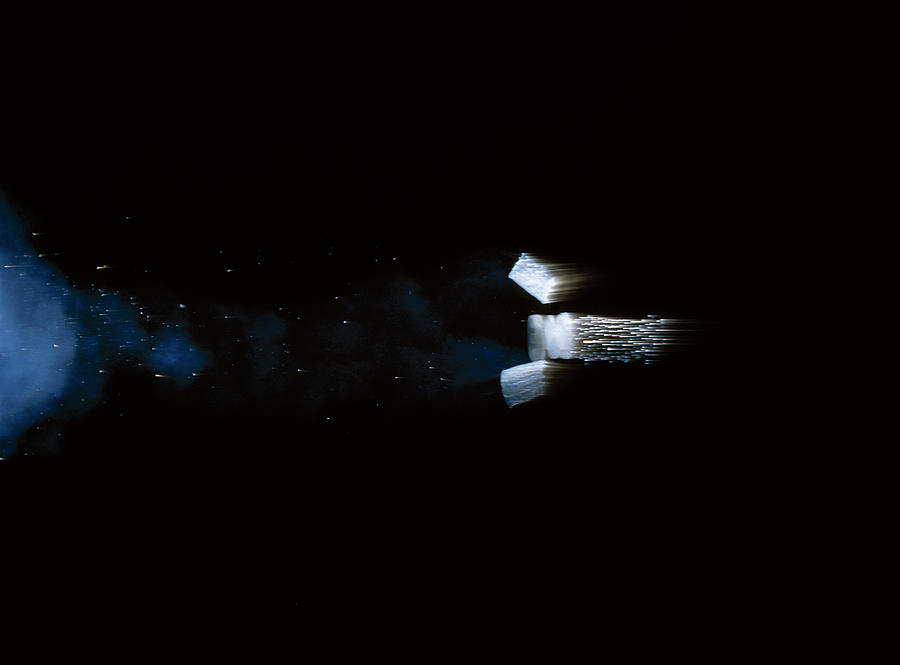This captivating and enigmatic image is a high-speed photograph set against an entirely black background, creating a stark and dramatic contrast. On the far left, a blue cloud of smoke or powder billows outward, spreading across the midsection of the picture. The central right portion of the image features three small, reflective cubes or squares from which white, silverish trails emerge, reminiscent of a firework. These trails are dotted with various colors, including gold, silver, and hints of purple, adding to the visually striking scene. The object or objects appear to be moving apart at high speed, leaving a trail of debris and powder-like particles. The surrounding space is dotted with white splotches, possibly stars or reflected remnants, enhancing the sense of motion and complexity in this mesmerizing and scientifically intriguing image.